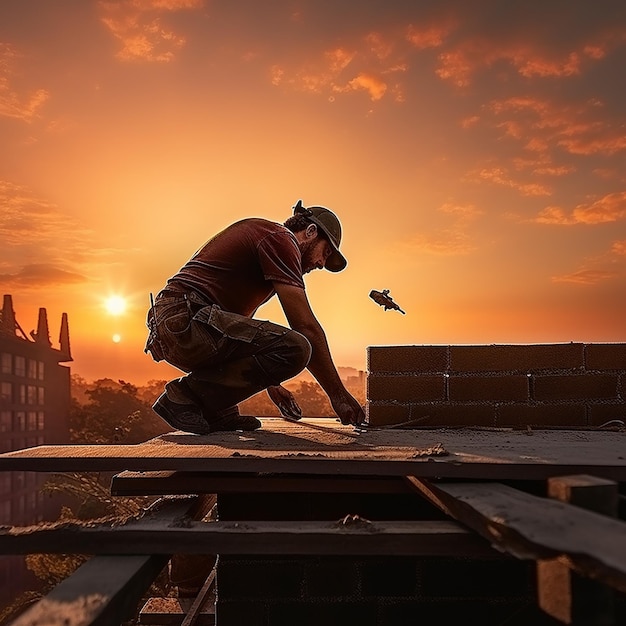In this vivid, sunset-lit image, a man is working on the roof of a high-rise building. The sky glows with a deep orange hue, with scattered clouds and both the sun setting and the moon rising in the background. The man, who is the central focus, is wearing a baseball cap, a dark brown t-shirt, and camouflage pants. He has a walkie-talkie clipped to his hip and appears to be measuring something. The rooftop is strewn with wooden boards and sections of potential scaffolding, exposing open areas that give a glimpse into the building below. In the sky, a helicopter is visible, adding a dynamic element to the serene, yet industrious scene set against an array of muted trees and a silhouette of a distant building. The blended tones of orange, black, and beige accentuate the overall atmosphere of concentrated effort at a transitional time of day.